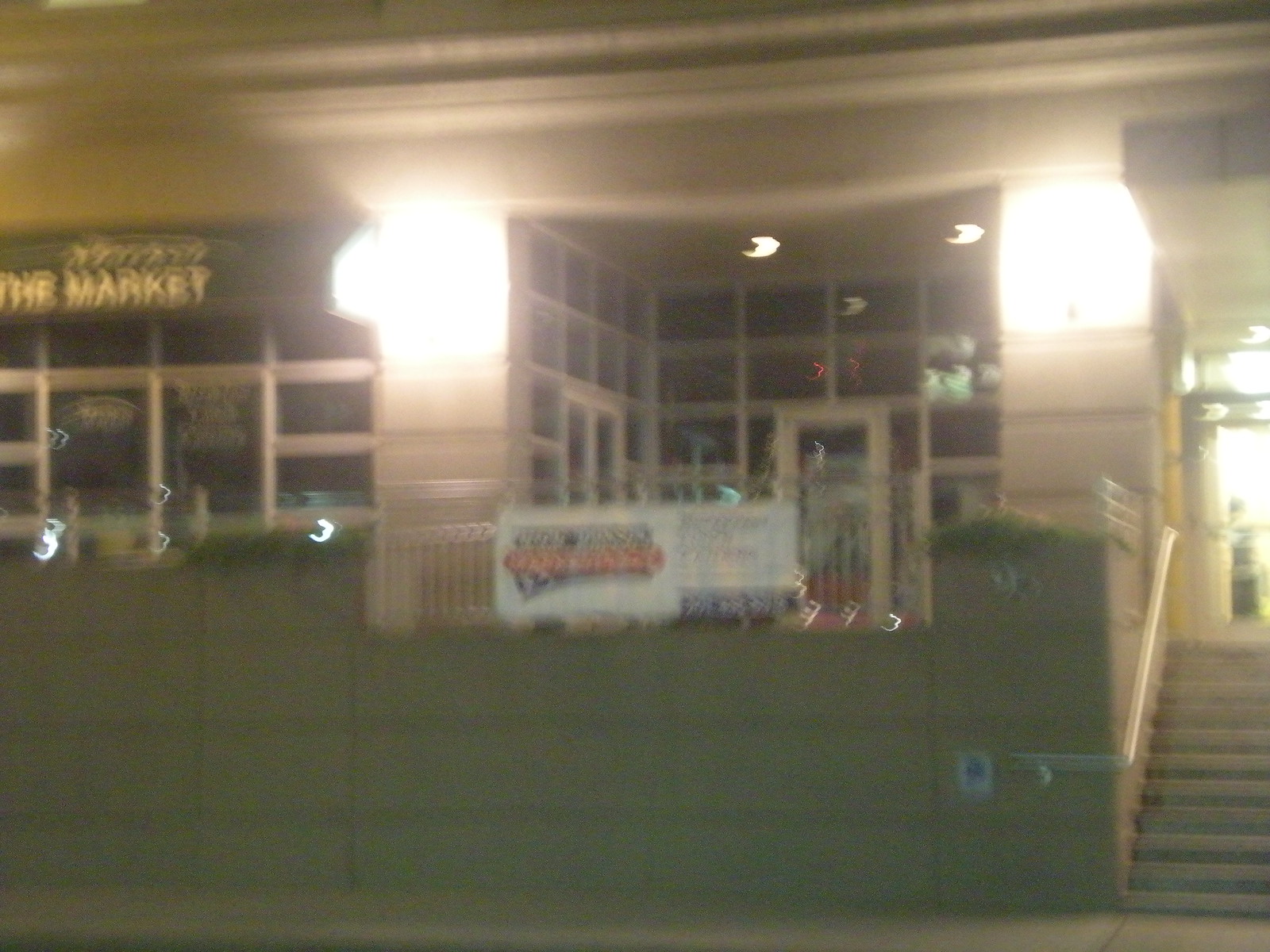Capturing the essence of a quiet evening, this blurry, low-quality photograph depicts the dimly lit exterior of a storefront, seemingly taken at night. The close-up shot emphasizes a small set of stairs situated on the lower right side, leading up to the entrance on an elevated level. To the left of these stairs, a partial view of a wall is visible, extending further to reveal two additional storefronts in the background. The leftmost storefront is partially cut off by the frame. Above the primary entrance of the main storefront, which features an all-glass facade, a green sign with gold lettering reads "The Market." The overall scene suggests that the stores are closed, as indicated by the absence of interior lighting and the tranquil nighttime ambiance.